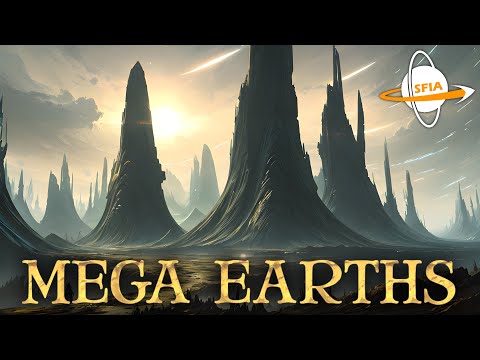The image portrays an otherworldly, futuristic sci-fi landscape dominated by surreal mountain peaks that rise into sharp spires, unlike anything found on Earth. The scene has a predominantly gray and brown color scheme with streaks of white, and the mountains are accentuated in green and brown hues. The sky above is a dramatic blend of blue and gray tones with a prominent yellow sunburst and wisps of golden clouds. The striking visual includes elements that add to its immersive quality: in the upper right corner, there's an emblem resembling a planet with small orange letters "SFIA" encircled by a yellow-orange line and a white arrow. Beneath this emblem is a white vertical ring. At the bottom of the image, framed by a solid black border, the title "MEGA EARTHS" is rendered in a fantasy-style gold font. The overall impression is that of a title image for a sci-fi game or audiobook, capturing a blend of awe-inspiring natural formations with an imaginative and speculative twist.